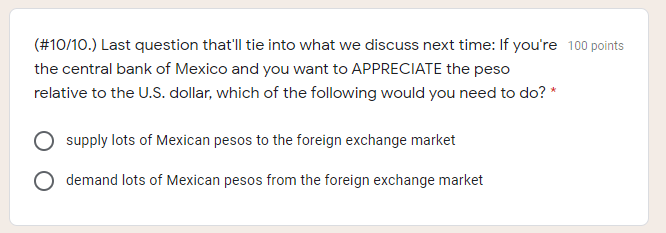An image showcases an educational slide focusing on a final question for a discussion session. The slide features a tan border and a white rectangular center. At the top, it is labeled "(10/10). Last question that’ll tie into what we discuss next time:", followed by the prompt: "If you’re the Central Bank of Mexico and you want to APPRECIATE the peso relative to the US dollar, which of the following would you need to do?". The word "APPRECIATE" is emphasized in all capital letters and there is a red star next to the question.

Below the prompt are two clickable options, each accompanied by a circle to indicate selection: 
1. "Supply lots of Mexican pesos to the foreign exchange market."
2. "Demand lots of Mexican pesos from the foreign exchange market."

Participants must choose the correct option by clicking on the corresponding circle, which will then display a check mark or blue dot to indicate their selection. The question is valued at 100 points.